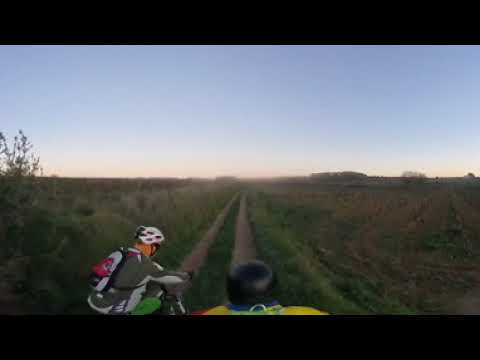The image portrays two people riding mountain bikes on a flat, dirt trail through a grassy, open field, under a clear blue sky with a setting sun. The trail features car tracks with a grassy strip down the middle. The person in the foreground is more visible; they are wearing a white helmet and a gray and lighter gray jacket, carrying a gray, black, and pink backpack, and riding a gray bike with white graphics. The second person, partially visible from the top, dons a black helmet and a brightly colored jacket featuring yellow, green, red, and blue elements. The photo has thick black rectangles framing the top and bottom, hinting at a cinematic style. The dirt path is brown, lined with stretches of green grass, embodying the serene yet adventurous spirit of the outdoor scene.